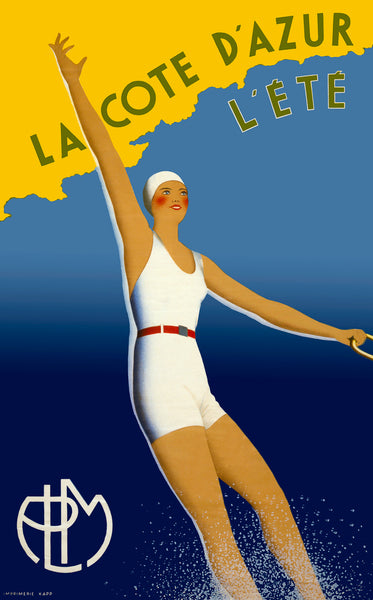The image is an eye-catching, digitally rendered poster depicting a woman swimming in a vibrant, vintage style reminiscent of older travel advertisements. At the center, a tanned woman with exaggerated limbs and a small head wears a one-piece swimsuit with a red belt and a white swimmer’s cap. Her right hand is raised towards the top left, while her left hand holds a gold ring horizontally positioned on the right side of the image. The woman is partially submerged in water, causing a dramatic white splash near her feet.

The backdrop features a coastal scene with a landmass in the top left corner. The water surrounding her transitions from light blue in the middle to darker blue at the bottom, complemented by splashes of yellow and tan accents, bringing a lively yet calming palette to the image.

At the top of the poster, there is a yellow area with a texture resembling a ripped surface. In this area, olive green text prominently states "La Côte d'Azur," followed by "L'Eté" in a bluish color. The bottom left corner showcases a white logo that seems to consist of the letters "PLM," although it is somewhat difficult to discern. The overall design is bright and clear, creating an inviting and nostalgic atmosphere reminiscent of a sunlit summer day on the French Riviera.